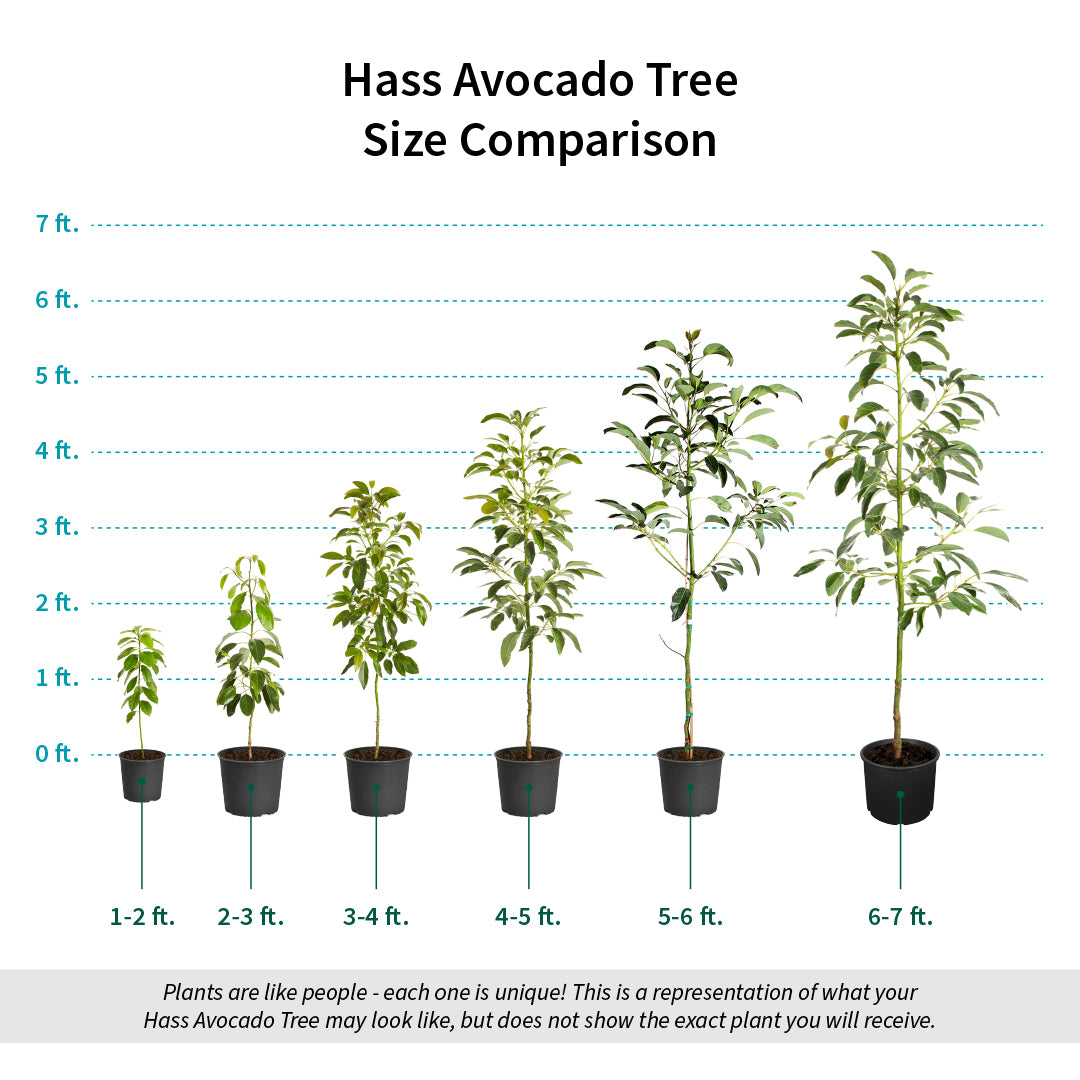The color infographic titled "Haas Avocado Tree Size Comparison" depicts six avocado trees of varying heights in black buckets. On the left side, a height chart marked in one-foot increments from 0 to 7 feet serves as a reference. The trees are arranged horizontally along the bottom, with labels indicating their respective sizes: 1-2 feet, 2-3 feet, 3-4 feet, 4-5 feet, 5-6 feet, and 6-7 feet. A gray band positioned below these labels features the text in black font, "Plants are like people, each one is unique. This is a representation of what your Haas avocado tree may look like, but does not show the exact plant you will receive." This detailed comparison offers visual guidance for potential buyers on the expected size variations of Haas avocado trees.